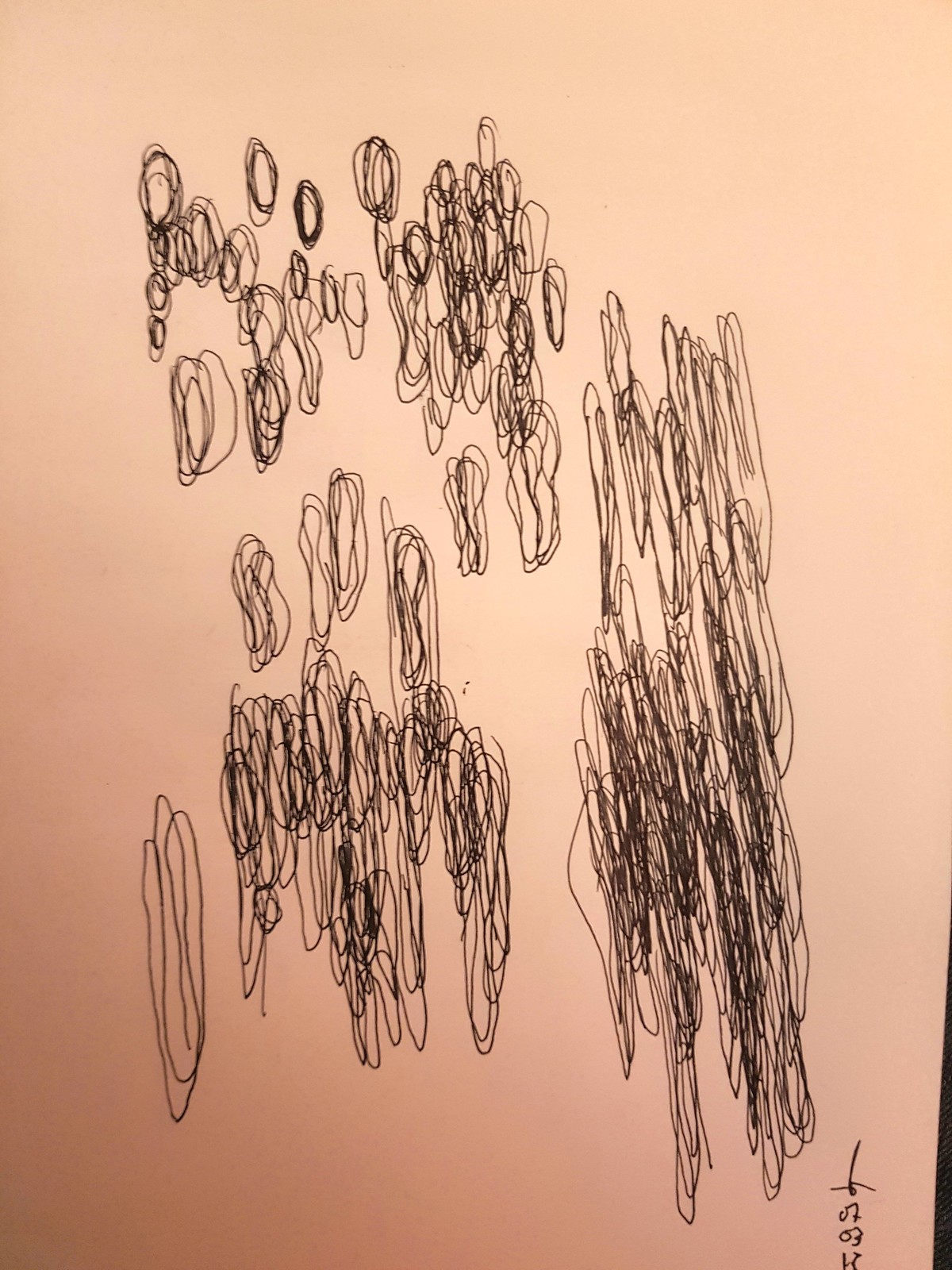The image features a long piece of pink paper, occupying most of the frame, with a sliver of a dark background visible at the bottom right corner. Along this dark edge, small, enigmatic numbers and symbols, including O2, O3, and a K, can be seen. The paper is heavily marked with black pen ink, characterized by an array of concentric circles, both large and small, haphazardly overlapping each other. These markings vary in intensity, some forming heavy, almost solid black scribbles, while others are lighter and more misshapen, resembling little spirals.

On the right side of the paper, there are dense, long, and thin pen strokes layered atop one another, gradually giving way to less concentrated, thinner marks. The chaotic interplay of thick and thin lines creates a textured and dynamic visual, with areas of densely packed ink contrasting against more sparsely drawn sections.